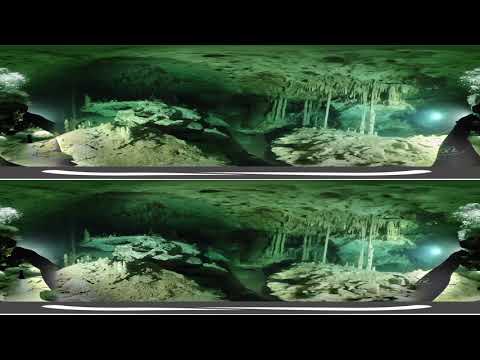The image comprises two stacked photos, seemingly taken at different times, of an underwater cave or cavernous area. The scene is predominantly tinted green, with traces of blue and hints of gray and teal. Both images show the same spot, characterized by an abundance of algae covering the rocks. The cave’s interior features prominent stalactites and stalagmites. In both photos, a diver dressed in black scuba gear is visible on the left side, subtly changing position—one picture shows the diver with a bent leg, while the other has the leg extended. The overall setting is dark and shadowy, resembling night vision imagery, and evokes a sense of eerie beauty despite its somewhat intimidating atmosphere. There are no fish or additional marine life visible, emphasizing the solitude and stillness of this underwater world.